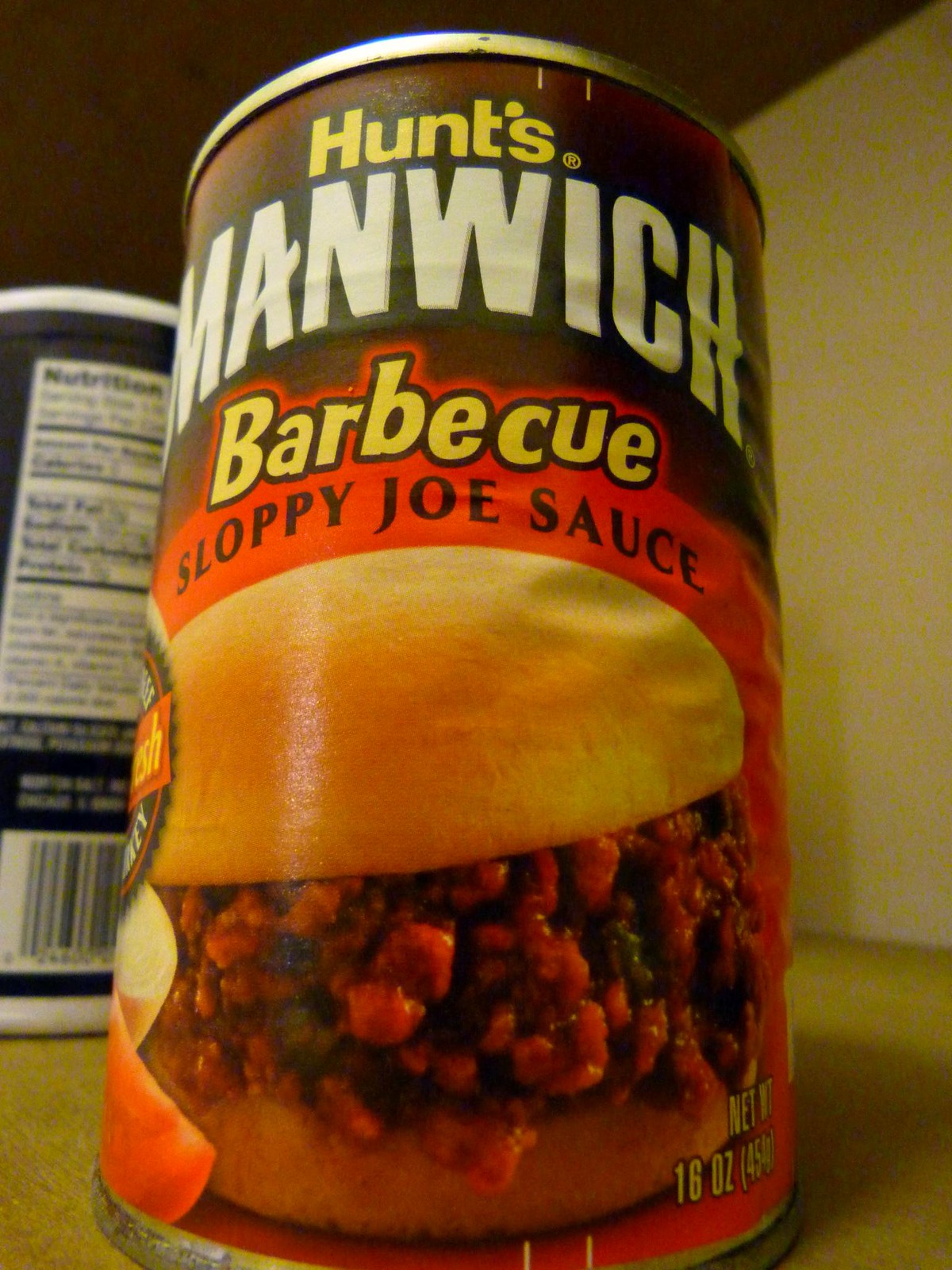This image showcases a close-up view of a can of Hunt's Manwich BBQ sloppy joe sauce, evoking a vintage aesthetic. The can's top is dull, lacking the shine of newer products, and the label itself appears worn with slightly bent edges. The label features a brown upper section with the word "Hunt's Manwich" prominently displayed, followed by a red section where "BBQ" is written in bold yellow print. The label also includes an appetizing image of a bun filled with the Manwich BBQ meat. In the background, the blurred outline of another container is visible, characterized by a white top and a dark navy blue or black label, though the specific branding remains unreadable. The overall photograph has an aged quality, further contributing to its vintage charm, with colors that are muted and a slightly faded appearance.